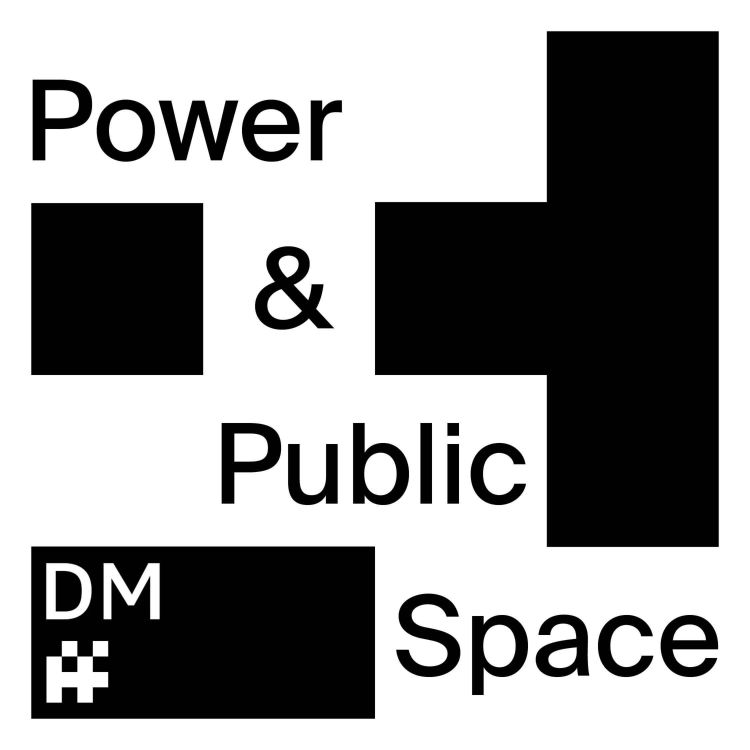The image is a black and white graphic design on a pure white background. It features text and geometric shapes that closely resemble Tetris blocks. The primary composition includes a sideways T shape made out of identically sized black squares on the right-hand side. This T shape consists of one square in the center, representing the bottom of the T, and three stacked squares extending to the right. To the left of the central square of the T, there is a small white square, followed by another black square of the same size. Two squares down, in the bottom left corner, there is a horizontal row of two black squares.

The text on the image is distributed within the white portions of the background and reads: "POWER & PUBLIC SPACE" in black letters, printed in a basic font that stretches from the top left to the bottom right. In the bottom left corner, embedded within a black shape, there is a white QR code-like design accompanied by the letters "DM" in white text.

Overall, the image offers a minimalistic yet striking visual composition, potentially hinting at themes related to social justice or public engagement.